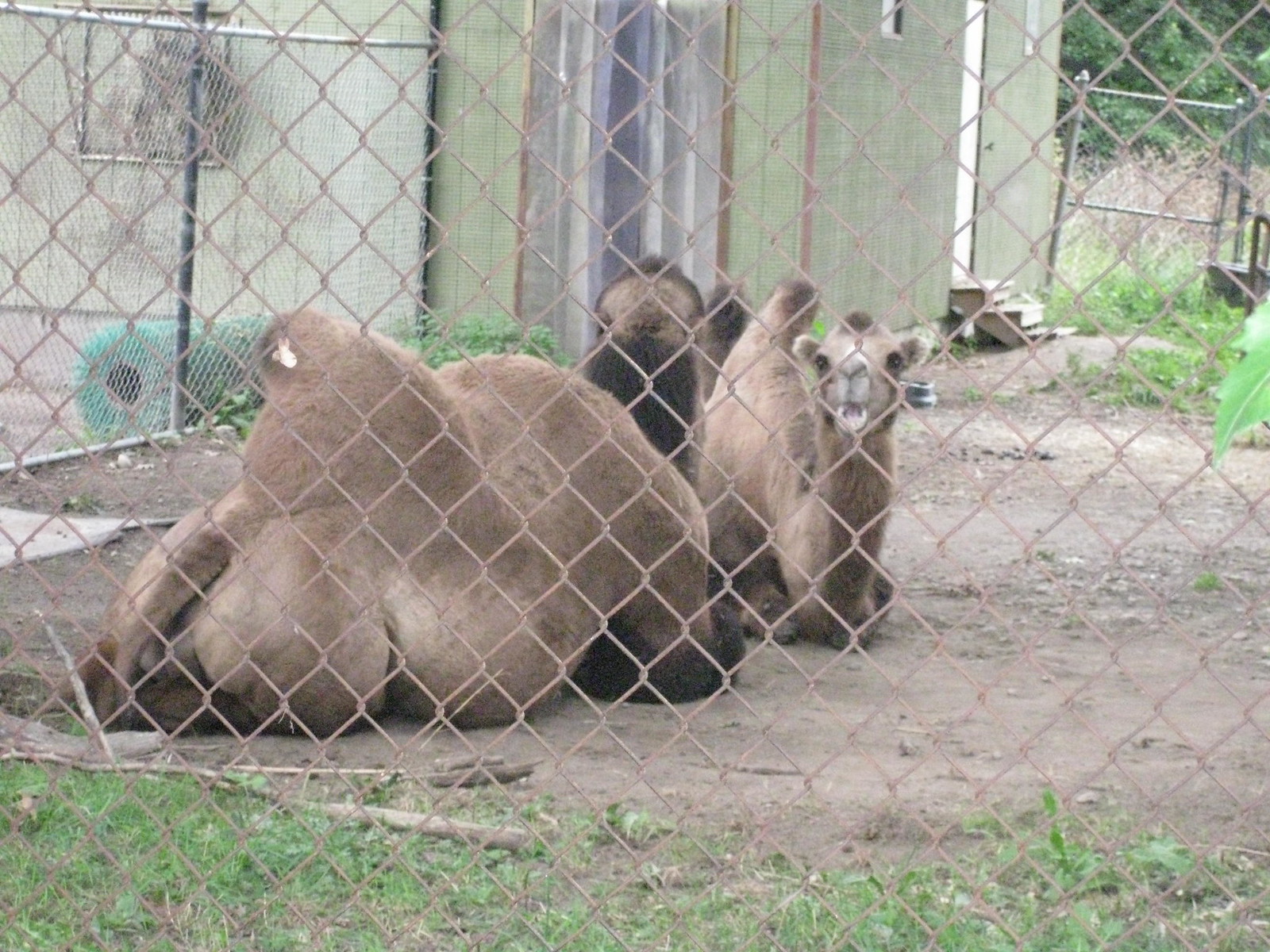In this slightly poor-quality color snapshot, taken during the day, three camels are lounging inside an enclosed, rusted chain-link fence that runs diagonally across the image. The ground is primarily light brown dirt with scattered patches of green grass. The central camel, which is smaller in perspective and looking directly at the viewer, has a mix of light brown, tan, and white fur with notably white markings on its face. This camel appears to have its mouth open in a peculiar, taco-like formation. Facing away from the viewer is a larger camel, showcasing its hump and part of its tail and back. Behind this central camel is the faint indication of a third camel lying down. The enclosure is set against a light green wooden building located at the back-left of the frame, which features a white door and stairs leading down. A rolled-up piece of greenish fabric is visible to the far left of the image.